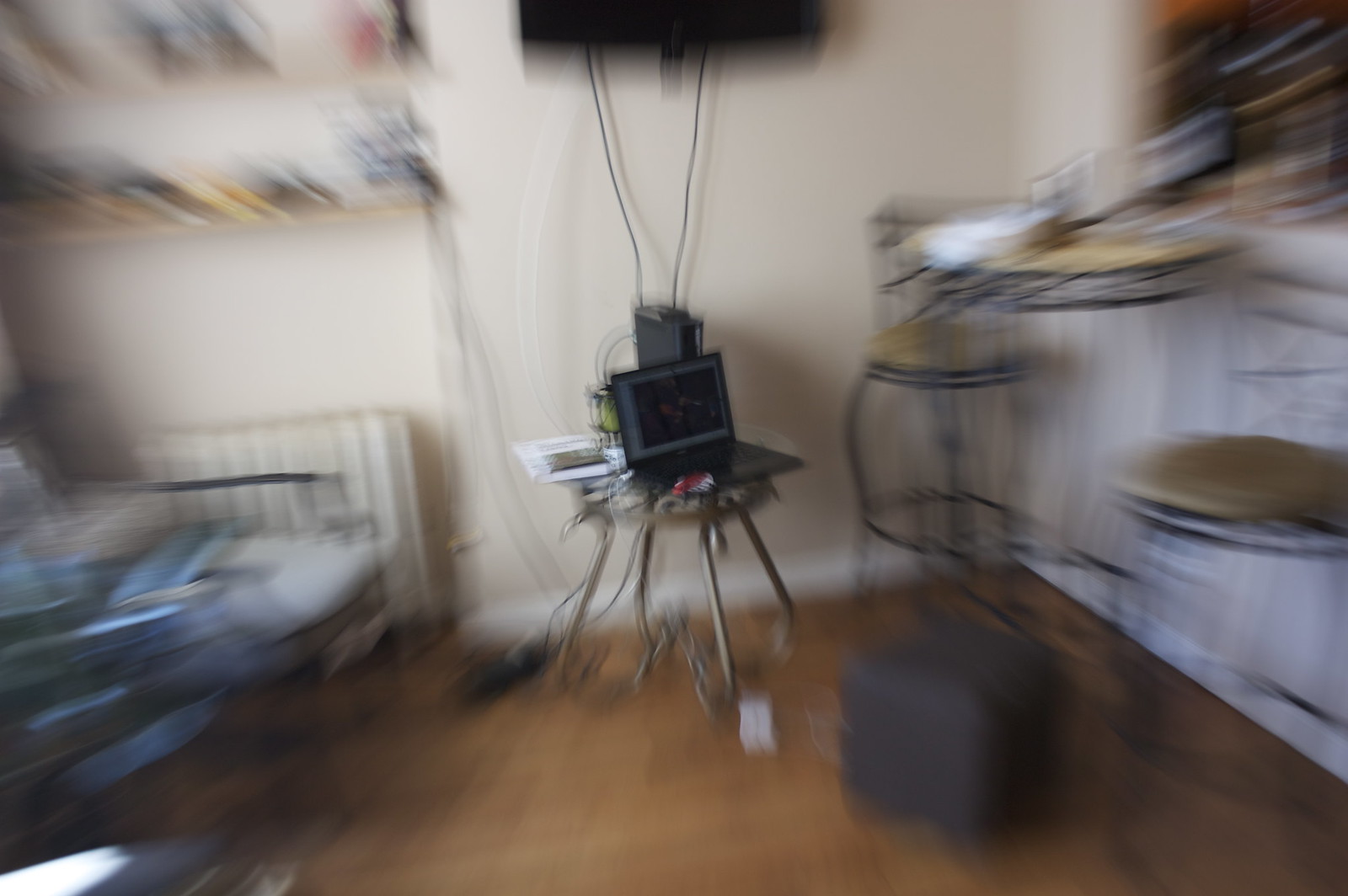In this blurred photograph, the focal point is a laptop positioned on a small, round glass table with elegant gold metal legs that curve downwards and meet at a central point. The background features a beige wall and white baseboards, with brown flooring beneath. On the right, there's a dark brown cube beside a stool with a gold top and black legs, and another matching stool further away, accompanied by a metal railing at the back. To the right, a white wall is visible, while the left side of the image reveals a shelving unit with wiring that likely connects to a black TV mounted above. An off-white heating element is affixed to the wall, and a bluish-grey object is partially visible on the left. Various other items, including what appears to be an electronic device with black cords, scattered books or papers, and additional undefined objects, contribute to the cluttered yet intriguingly detailed scene.